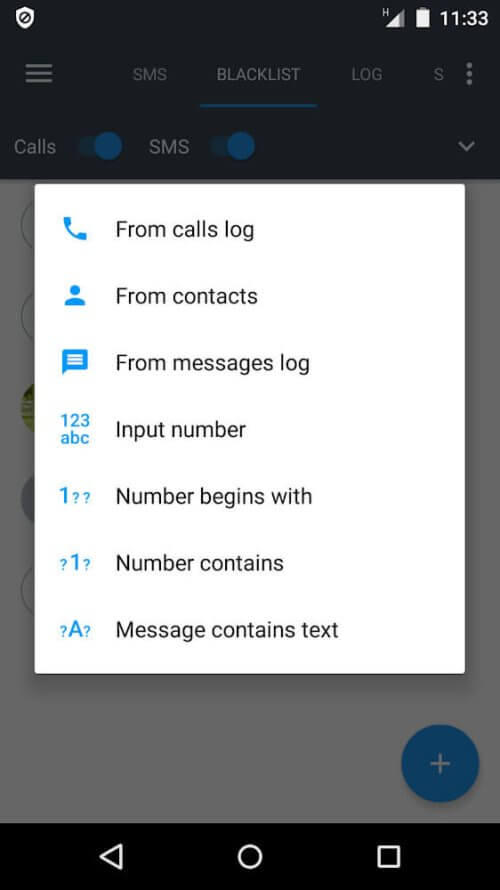A detailed screenshot of a smartphone displaying the "Blacklist" menu, suggesting it is set to manage blocked calls or messages. The top of the screen features typical interface elements such as signal strength icons, Wi-Fi connectivity, and the current time, all displayed in white font against a black background. The selected "Blacklist" category is highlighted at the top, alongside other options like SMS, Log, and specific filters for Calls or SMS.

Prominently, the "Blacklist" section is expanded, revealing further functionalities. On the left side, various icons indicate different sources: a phone icon labeled "From Calls Log," a blue contact icon labeled "From Contacts," a speech bubble icon labeled "From Messages Log," and a "123ABC" text input icon labeled "Input Number." 

Below these options are specific filters presented as lines of text that allow detailed customization of blocked entries. These include options like "Number begins with," "Number contains," and "Message contains text," each accompanied by placeholder symbols (e.g., question marks) indicating inputs or queries. At the bottom of this settings interface, standard control icons for play, stop, and window management provide additional navigation capabilities.

This comprehensive screenshot provides a clear overview of how the phone is configured to manage unwanted communications through its blacklist feature.